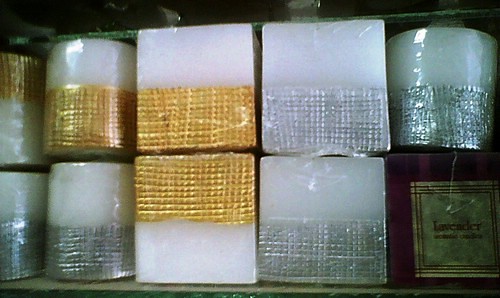The image shows a neatly arranged collection of nine candles displayed on a glass shelf with minimal spacing between the levels. At the bottom, there are two circular white candles, each adorned with a decorative silver foil pattern at the base, creating an elegant contrast. Above them sits a second row, featuring a pair of square candles; the upper square candle has gold foil on top and white on the bottom, while the lower one has the gold foil pattern at the base. The upper layer mirrors the pattern of the lower layers: first, a circular white candle with a gold foil bottom, then another circular candle with a silver foil bottom. Concluding the collection, a dark brown square candle with a green interior can be seen in the upper right corner, adding a touch of color variety to the display. Each candle provides a harmonious blend of white, gold, and silver, further accentuated by patterns etched into the foil wrappings.